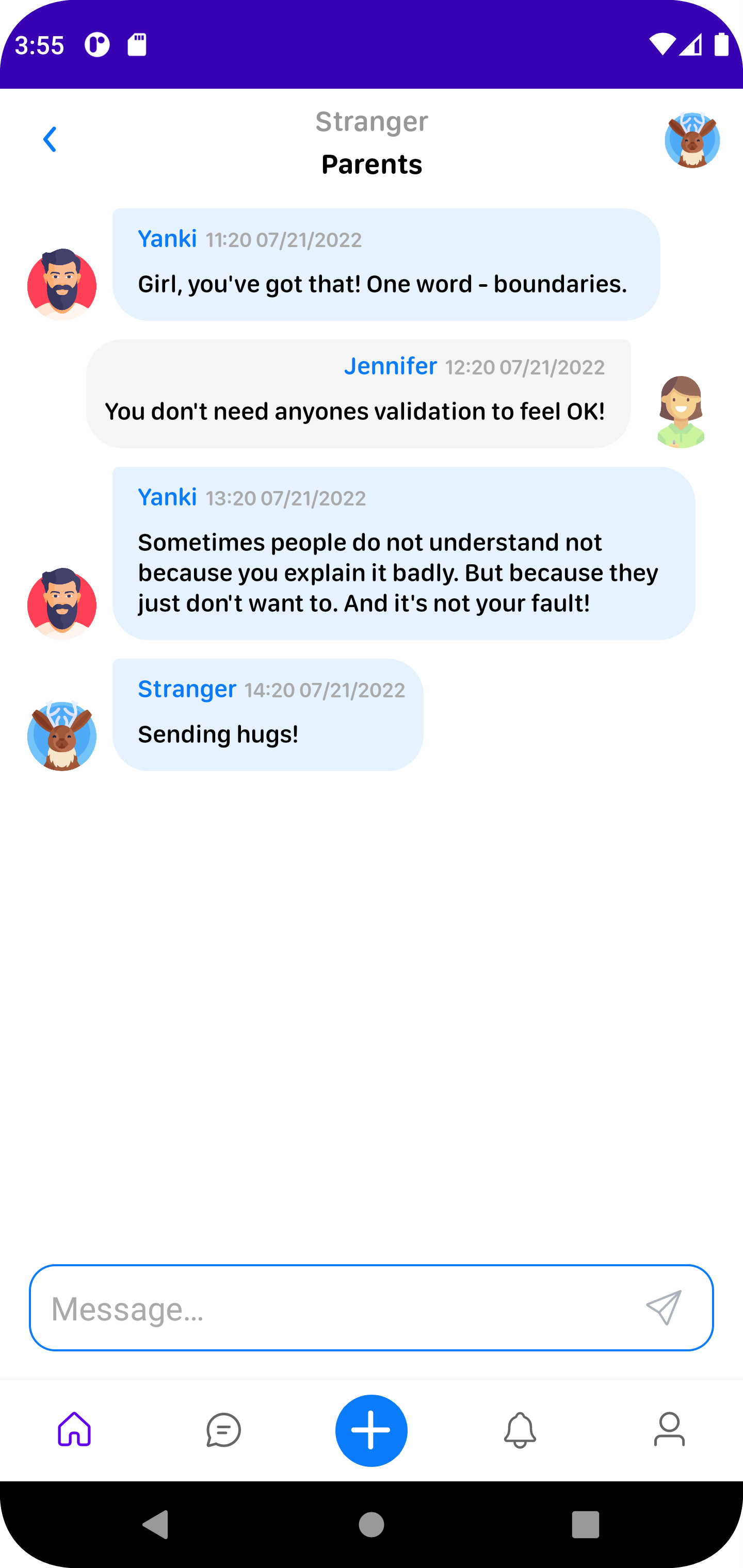A smartphone screen displays an active instant messaging conversation with a detailed interface. At the very top, a banner features a blue background that includes the current time "3:55," a small "R" logo next to a document icon, and various status icons like battery life. The conversation is housed within a white background, where different dialogue boxes alternate between gray and light blue.

A message appears from "Yankee" in a blue box, stating, "Sometimes people don't understand that, not because you explain it badly, but because they just don't want to. It's not your fault." This follows an earlier message from "Jennifer" in a gray box, advising, "You don't need any validation to feel okay." Another blue box from "Yankee" sends encouragement: "Sending hugs."

The labels "stranger" in gray and "parents" in bold text are observed in the interface, indicating different participants in the conversation. Additionally, the interface includes various controls and options at the bottom: a blue-bordered text input box with a send button, a home icon, a text icon, a plus sign within a blue circle, an alert icon, and a person icon. At the very bottom, the navigation bar features a back arrow, a solid circle, and a square.

The composition accurately captures an ongoing supportive and heartfelt exchange, emphasizing themes of understanding and mutual encouragement amidst an intricate and well-designed messaging interface.